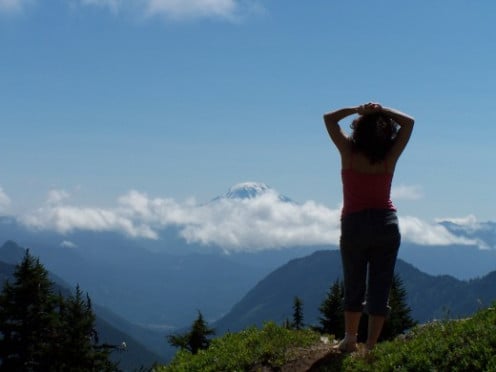A woman stands barefoot on a grassy, dirt path atop a mountain, facing away from the camera. Her medium-length dark hair rests on her back, and she wears a red or pink tank top with thin straps and cropped blue pants, rolled up halfway up her calves. Both her arms are stretched overhead with her fingers interlocked, as she looks out towards a breathtaking panorama of mountains. The scene is described under a bright, light blue sky dotted with fluffy white clouds, suggesting a clear, sunny day. In the distance, various mountain ranges extend for miles, with a snow-capped peak visible in the far background. The woman stands notably above the line of pine trees, which flank the sides and foreground, marveling at the expansive natural beauty before her.